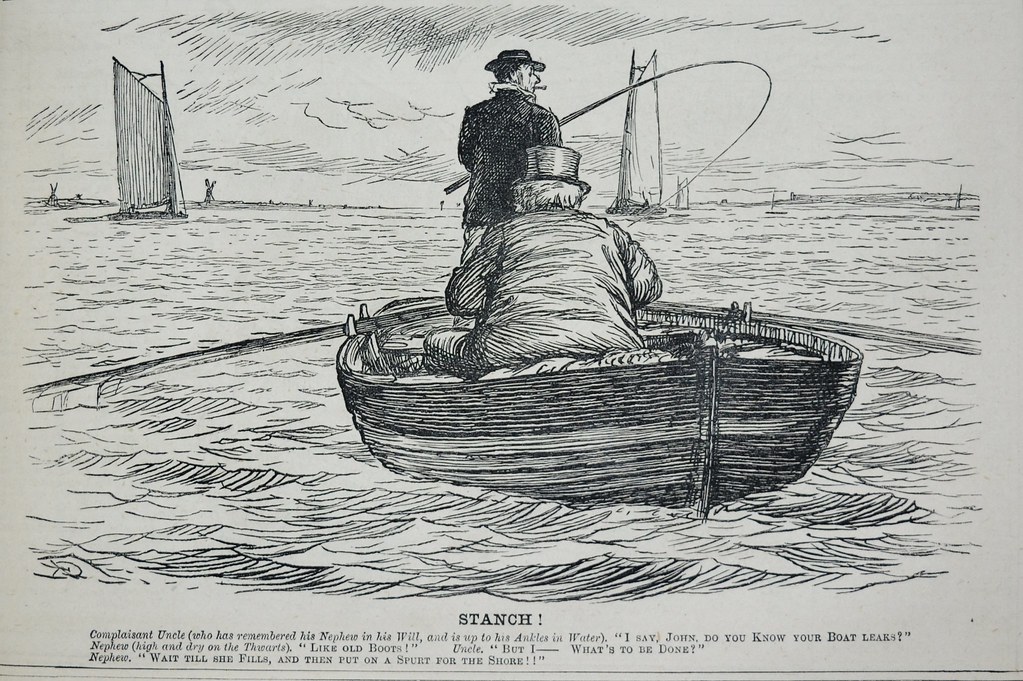The image is a black and white, hand-drawn, landscape layout cartoon, primarily depicting a scene on the water. Most of the composition is filled with water, with minimal sky above, drawn with lines representing clouds. The central focus of the artwork is a rowing boat, viewed from the back. In the boat, two men dressed in suits are present. One man, seated and rowing, has his back to the viewer and wears a top hat. The other man, standing at the front and facing sideways, holds a fishing rod or a whip, has a hat on, and a cigarette in his mouth. In the distance, two additional sailboats are visible. The bottom of the image contains bold black text stating "STAUNCH!" along with other smaller text, suggesting the image might be a political cartoon. Additionally, there is some annotation in small print, possibly adding context or a punchline to the artwork, which appears to be set in the 1800s.